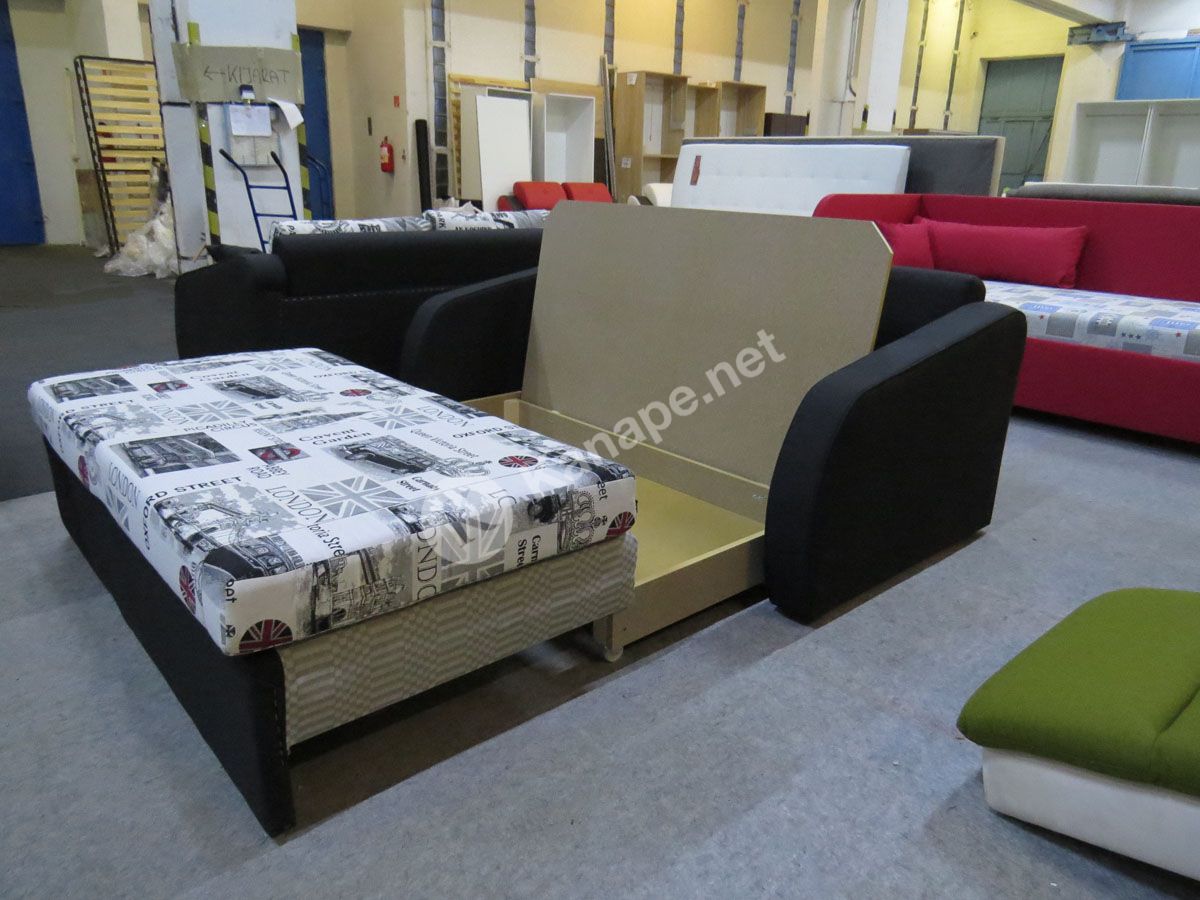In the image, the center focus is a black loveseat that folds out into a bed, situated in a furniture showroom. The loveseat features a unique newspaper or comic book-themed fitted bedsheet over a small mattress, offering both a stylish and functional appeal. The bed's foot is angled to the left, with the black frame complemented by a beige baseboard. Beneath the mattress is a dark gray box spring, and the couch arms are large and round. The loveseat includes a compartment at the back that flips up to store the mattress when converted back to a couch. The backdrop showcases a spacious, white-walled showroom lined with various pieces of furniture, including an identical loveseat in red to the right, and another to the left. The bottom right corner reveals a partially visible green lounge chair with a white base. A watermark reading "Hanepe.net" is noticeable, alongside assorted furniture items like wooden bookcases without shelves and a hand truck in the distant background, enhancing the setting's authenticity.